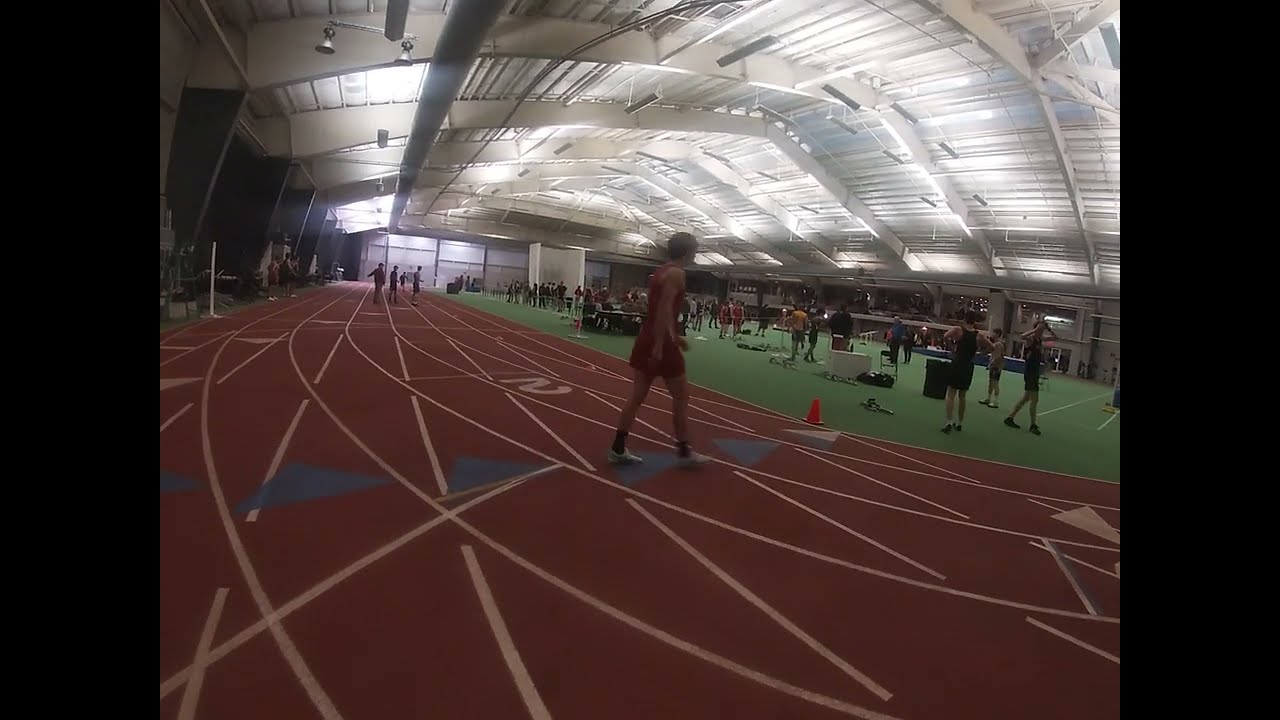This image depicts an indoor track field within a large facility characterized by overhead lighting and concrete reinforcements. The scene appears to be part of a gymnasium, potentially at a high school, evidenced by the surroundings and attire of the individuals present. There are black borders on both sides of the image, suggesting it might be a screenshot from a video.

In the center of the image, a person dressed in a red track uniform, consisting of a red short sleeve shirt or tank top and red shorts, is prominently featured. They are walking towards the middle of the track area, rather than running, drawing clear attention to their presence. The track itself is colored in a dark red or brown shade, marked by white lines and blue directional arrows to guide runners.

To the left side of the image, the visually striking track lanes are visible, complete with numbered lanes and markers to maintain order during races. On the right side, there is an area covered in astroturf or artificial green, where several other individuals in track or sports uniforms are gathered. Among them, some appear to be setting up or interacting around a net, possibly for playing volleyball or badminton, adding to the multifunctional use of the space.

In the background, additional sports equipment is visible against the wall, enhancing the athletic environment and reflecting the facility's comprehensive setup for various indoor sports activities. The overall scene captures a moment of preparation and movement, rather than an ongoing race, providing a dynamic yet organized snapshot of indoor track and field life.